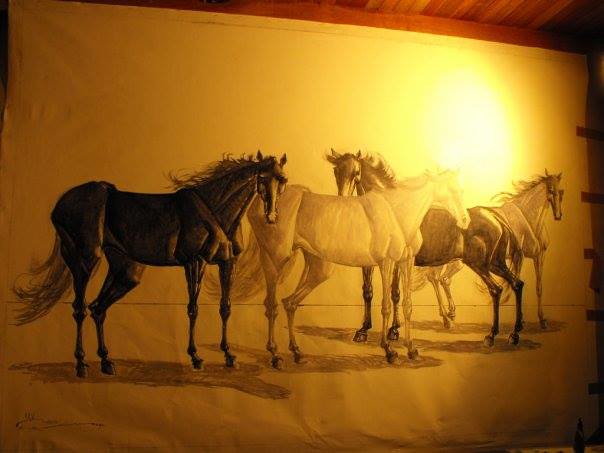This detailed art piece depicts four horses masterfully drawn in pencil on a white canvas, set against a wooden background. The composition is monochromatic, utilizing varying shades of black, white, and gray. On the far left, there is an intensely dark black horse facing to the right. Adjacent to it is a white horse that slightly overlaps with the horse behind it. This overlapping horse, a lighter black, faces to the left. On the far right, there is a gray horse, also facing right. Each horse casts pencil-drawn shadows that enhance the depth of the image. Above the third and fourth horses, there is a pronounced bright light or reflection that adds a dynamic element to the scene, suggesting a flash or some intense source of light shining from above. The meticulous pencil work brings life to this compelling portrayal of horses in motion.